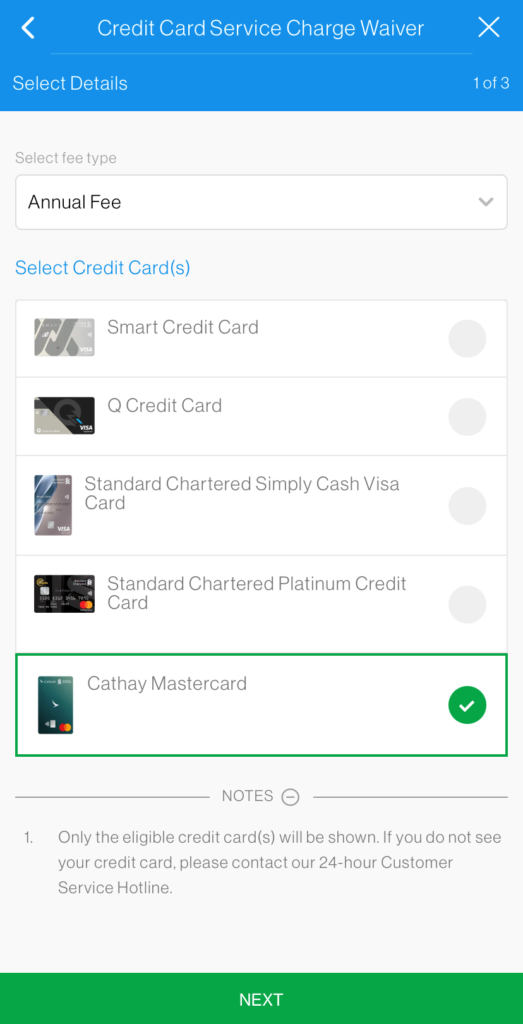The screenshot depicts a user interface from a mobile device showcasing a credit card service change waiver. At the top of the screen, the title "Credit Card Service Change Waiver" is prominently displayed. On the left side, there's an arrow indicating navigation, while the top right corner features an 'X' for closing the screen. Directly below the title, a prompt reads "Select details, one of three." 

The interface presents various credit card options. The "Annual Fee" section is followed by a list under "Select Credit Cards," which includes: Smart Credit Card, Q or O Credit Card, Standard Chartered Simply Cash Visa Card, and Standard Chartered Platinum Credit Card. Each of these options is accompanied by an unchecked gray circle.

Highlighted among these choices is the "Cat Hay MasterCard," set within a green rectangle and marked with a green check mark to its right, signifying its selection.

Further down, on a light gray background, there's a "Notes" section centered on the screen with two points:
1. Only eligible credit cards will be shown.
2. If you do not use your credit card, please contact our 24-hour customer service hotline.

At the very bottom of the image, a green rectangle button labeled "Next" in white text invites the user to proceed to the next step.